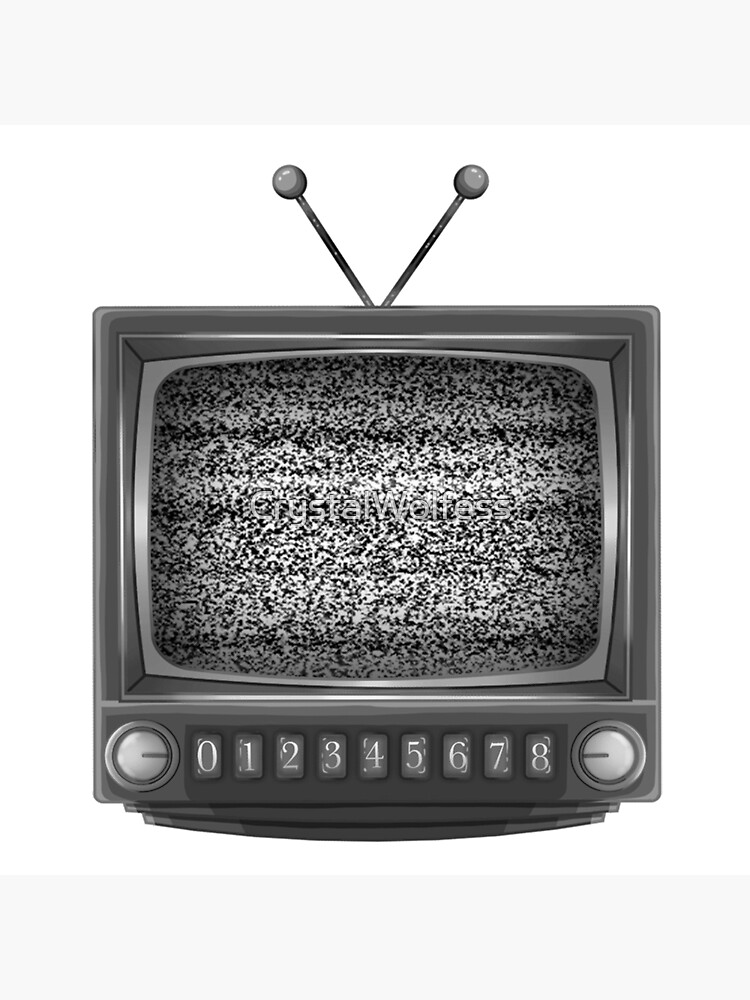The image depicts a classic vintage TV box rendered in black and white. Its square body features an oval-shaped screen filled with static, with faint, barely discernible text across the display that might read "Crystal Wolf" or similar. Prominently rising from the top middle of the TV are dual V-shaped antennas capped with small spheres. Below the screen, the TV boasts a switch panel with two control knobs on either side, likely for power and volume adjustment. Between these knobs are numbered buttons labeled from 0 through 8, hinting at the limited channels available on this retro device. The TV sits atop a slightly curved, two-layer base, adding to its old-school charm.